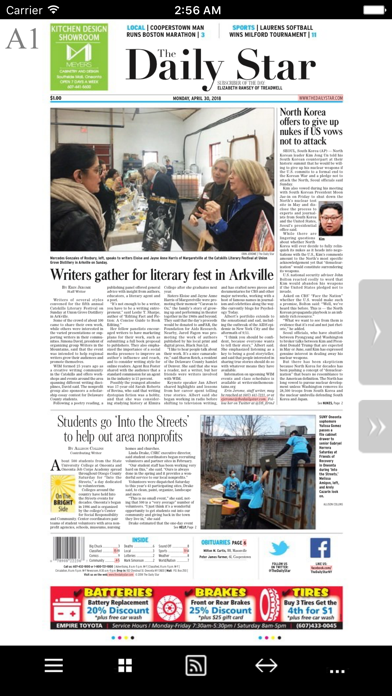The newspaper displayed on the phone screen shows various elements. In the top left corner of the phone's interface, it reads 'Carrier,' followed by a connection symbol and the time '2:56 AM.' At the top left of the newspaper article, the section is labeled 'A1.' There's a green box containing the text 'Kitchen Design Showroom,' accompanied by a logo and much smaller, unreadable text. 

Centered at the top, the newspaper's title 'The Daily Star' is prominently displayed, flanked by small, unreadable text above and below it. Below the title, a candid photograph captures several women gathered in a hall, engaged in conversation. The caption below the image states, 'Writers gather for literary fest in Arkville.'

To the right, there is another headline: 'North Korea offers to give up nukes if U.S. vows not to attack,' which includes a small embedded image of Kim Jong-un. Below this article, another headline reads, 'Students go into the streets to help out area non-profits.' The accompanying photograph shows students wearing blue shirts, most likely representing an organization, seemingly engaged in community service or clean-up activities, though the exact nature of their work is unclear.